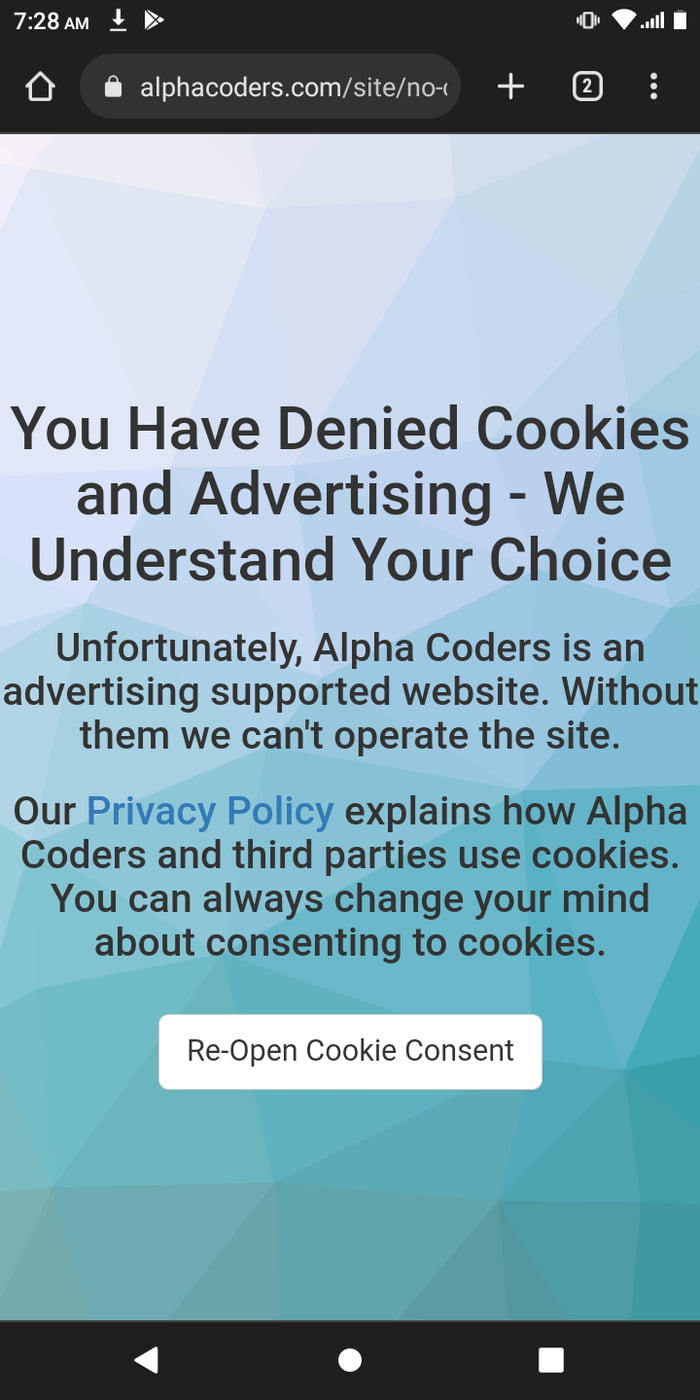Screenshot Description:

At the top of the image, there is a black banner with white text displaying "7:28 a.m." along with a Wi-Fi icon, a battery icon, and a vibration mode icon. Below this, there's an arrow icon with a line beneath it, followed by the Google Play Store icon. The website visible on the screen is AlphaCoders.com, indicated by a white house icon and a padlock symbol in the address bar. Next to this, there's a white plus sign and a square box with a white number "2" inside, accompanied by three vertical white dots.

The background of the image features a geometric pattern in various shades of blue, including lighter blues, grays, and greenish blues. The main text on the screen, written in black font, states: "You have denied cookies and advertising. We understand your choice. Unfortunately, Alpha Coders is an advertising-supported website. Without them, we can't operate the site. Our Privacy Policy," with "Privacy Policy" highlighted in blue, "explains how Alpha Coders and third parties use cookies. You can always change your mind about consenting to cookies." Below this text, there's a white box with black font reading "Reopen Cookie Consent."

At the bottom of the image is another black bar displaying three icons: a white triangle, a white circle, and a white square. The image is characterized by excellent, large, easy-to-read font and crystal-clear image quality, with no other objects of note present.